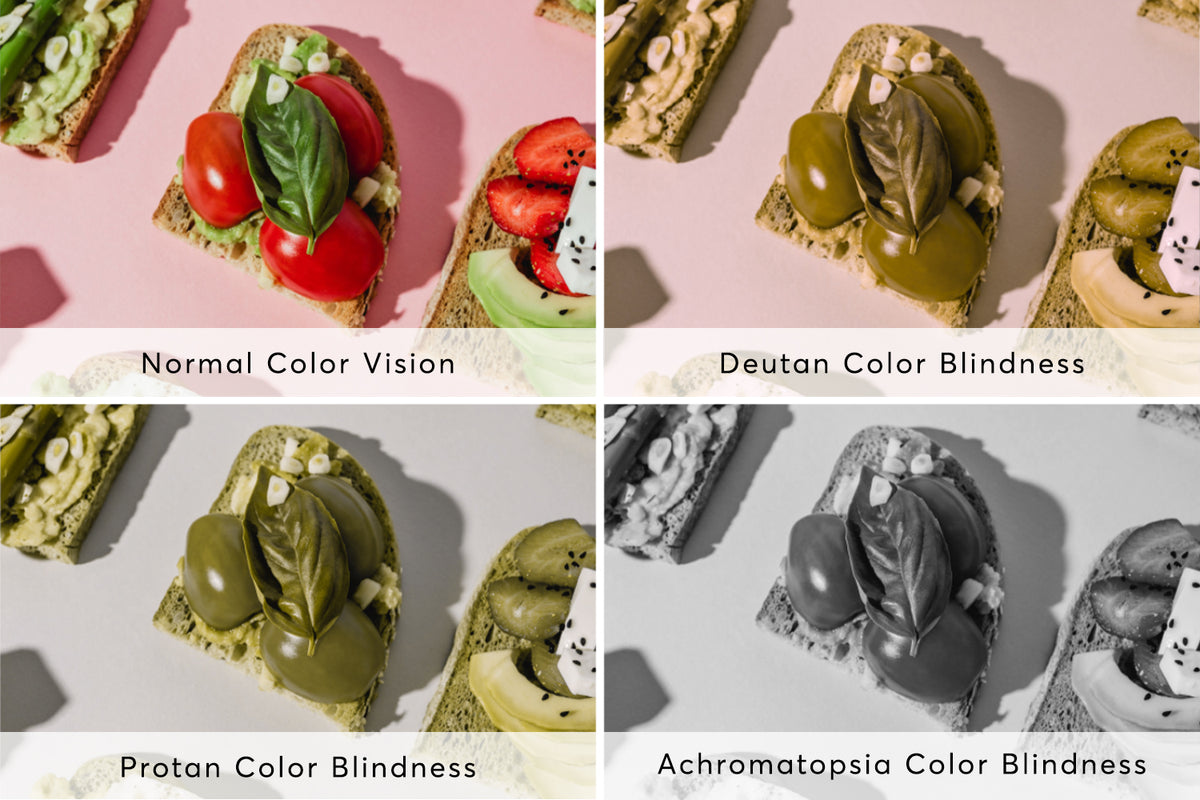The image is divided into four equal sections, each with a rectangular frame separated by white borders. In the upper left section, labeled "normal color vision," there is a small piece of bread topped with mozzarella, red tomatoes, and a green basil leaf. The background is bright pink, and the colors are vivid and true to life with the bread appearing brownish. To the upper right, labeled "Deutan color blindness," the same bread with toppings appears, but the colors have shifted to various shades of green. The lower left section, labeled "Protan color blindness," similarly displays the food, but in darker shades of green. Finally, in the lower right section, labeled "Acromatopsia color blindness," the image appears in black and white, devoid of any color. All four images depict the same composition of a piece of bread with various toppings to illustrate how different types of color blindness affect color perception.